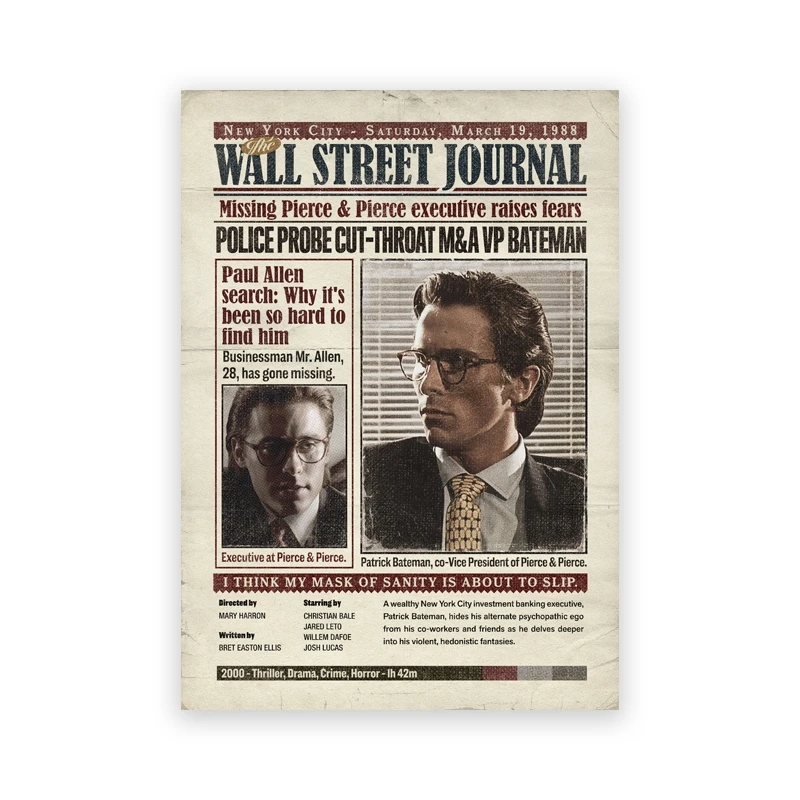This image mimics the front page of The Wall Street Journal and serves as an advertisement for the movie "American Psycho." At the top, there's a brown rectangular box with white text indicating "New York City, Saturday, March 19, 1988." Beneath this, "The Wall Street Journal" is displayed prominently in large black text. Below the headline reads, “Missing Pierce and Pierce Executive Raises Fears. Police Probe Cutthroat M&A VP Bateman."

Central to the image are two photographs. The one on the left features a man wearing glasses and a business suit, labeled "Paul Allen search: Why it's been so hard to find him. Businessman Mr. Allen, 28, has gone missing." The right-hand image, slightly larger, depicts another man in similar attire, but with a noticeable yellow tie. This caption identifies him as "Patrick Bateman, co-vice president of Pierce and Pierce." Both men appear quite similar, with short brown hair and glasses.

A quote beneath the images states, "I think my mask of sanity is about to slip." Towards the bottom, the film's production details are noted: “Directed by Mary Harron, Written by Bret Easton Ellis,” followed by “2000 thriller, drama, crime, horror - 1 hour 42 minutes." The page also features artificial wrinkles, rips, and tears, emphasizing its vintage look as part of the movie's promotional design.